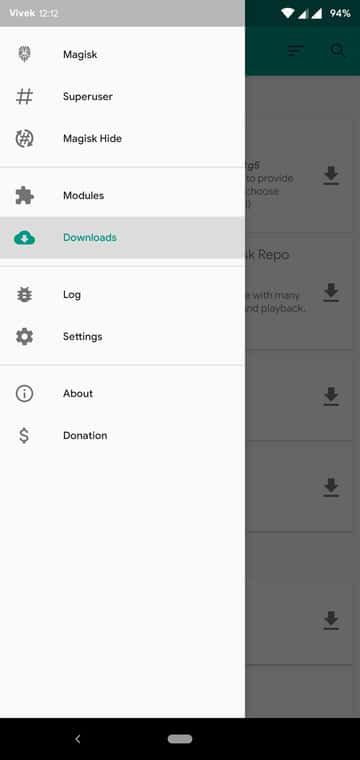The image displays a vertically elongated screenshot of a smartphone screen, approximately three times as tall as it is wide. In the upper right corner, standard status icons are visible, including two distinct Wi-Fi connections, a cellular signal indicator, and a battery status showing 94%, all in white.

Occupying about two-thirds of the screen on the left side is a slide-out menu from the active application. The menu has a predominantly white background, except for the top section, which is gray and features the text "Vivec 12.12" in white.

Within the white area below, several navigation icons and their labels are listed along the left edge. These options include:

1. Magisk
2. Superuser
3. Magisk Hide
4. Modules
5. Downloads

The "Downloads" option, located approximately 40% down the list, is highlighted, indicated by a gray bar extending horizontally across the menu item. The word "Downloads" and its associated cloud icon are both in teal. Further down the list, additional options such as Logs, Settings, About, and Donation are visible but not selected.

Overall, the image provides a detailed view of the menu structure within a specific app, showcasing both navigation and status information.